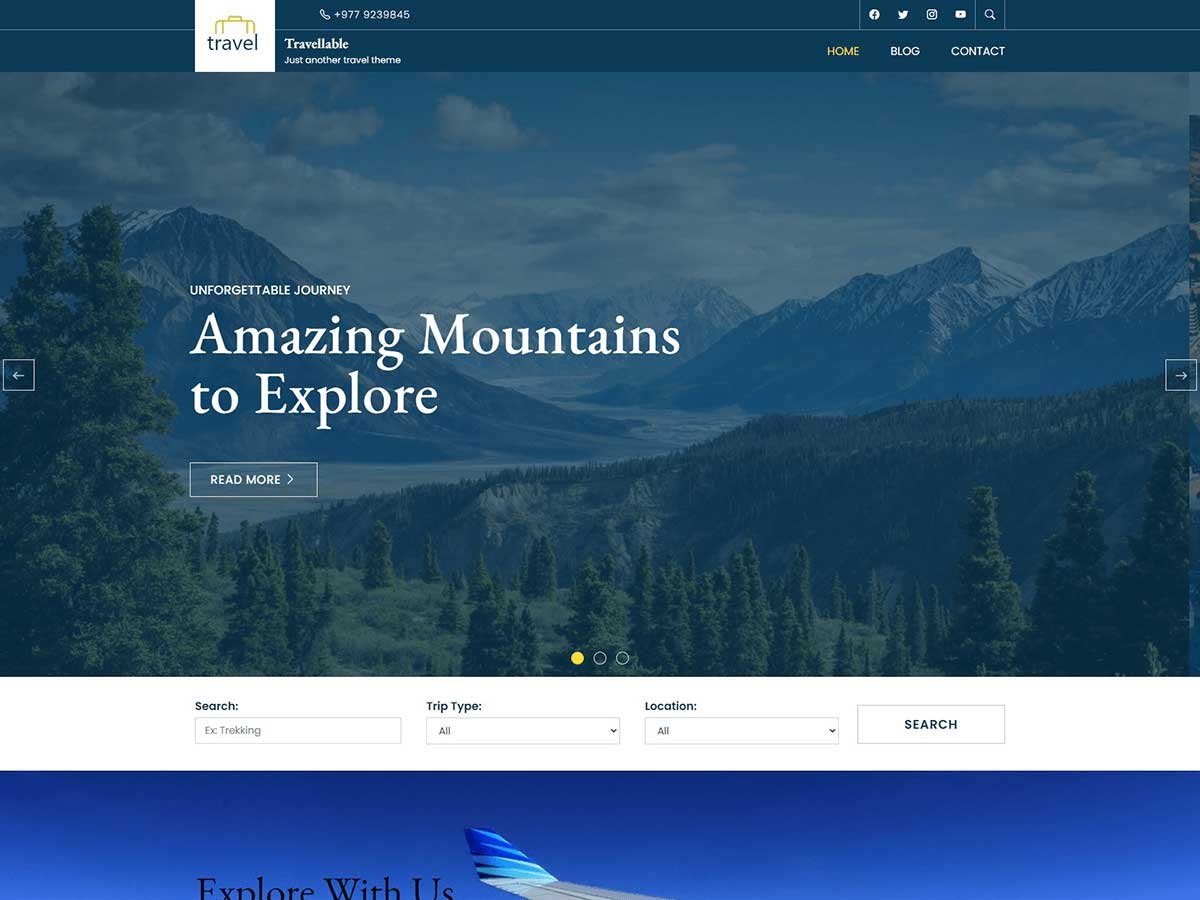**Detailed Caption:**

The image features a white page with a dark blue bezel at the top. Dominating the visual is a picturesque scene of dark blue mountains interspersed with patches of white, indicative of snow or mist. A river cascades down from these mountains, continuing through another range and onto a hillside. The landscape on the left and right sides is adorned with dense, dark green trees, with the right side appearing more densely forested.

A notable feature is a mountain ridge that stands out in gray. The entire image carries a blue hue, a result of a blue overlay that seems to blanket the scene. Prominently, there is a white arrow inside a square positioned centrally to the right of the image, mirrored by another on the left-hand side.

Central to this azure-hued image are the words "Unforgettable Journey," rendered in bold white text. Below, in larger font and also in bold white, the caption reads, "Amazing Mountains to Explore." Accompanying this text is a clickable button, rectangular with a blue border and a see-through or dark blue interior, bearing the bold white text "READ MORE" in all caps alongside a right-pointing arrow.

At the top of the image, within the dark blue bezel, there is a white square containing an off-green or gold briefcase icon, labeled with the bold blue word "TRAVEL," although the icon is partly obscured by the text. To the right, the phone number "+977 9239845" is displayed, and beneath it, "TRAVELABLE" (spelled out clearly) in bold white, followed by the phrase "just another travel theme."

On the right, navigation options include "Home," "Blog," and "Contact," with "Home" highlighted in yellow, indicating it is currently selected. The options "Blog" and "Contact" are displayed in bold white. Above these are the social media icons for Facebook, Twitter, Instagram, and YouTube, next to a magnifying glass icon for search functionality.

The bottom bezel of the image includes varied rectangular sections. One section features dark blue text "EX...TRACKING." Another section labeled "Trip Type" in blue includes a dropdown menu bordered in black with a white interior, displaying the text "FOR ALL" in bold. The "Location" field, also in dark blue text, has a white center with black text stating "THIS IS ALL" and includes a similar dropdown menu. A search button, white with a black border and dark blue text reading "SEARCH," is situated outside these sections.

Lastly, the scene includes the tip of an airplane, painted gray with bands of dark blue, cyan, and teal, flying under a dark blue sky with white bands. The left side partially displays the phrase "EXPLORE WITH US," though it is cut off.

This image encapsulates a compelling call to adventure, inviting viewers to delve into the majestic mountains and multifaceted travel opportunities provided.